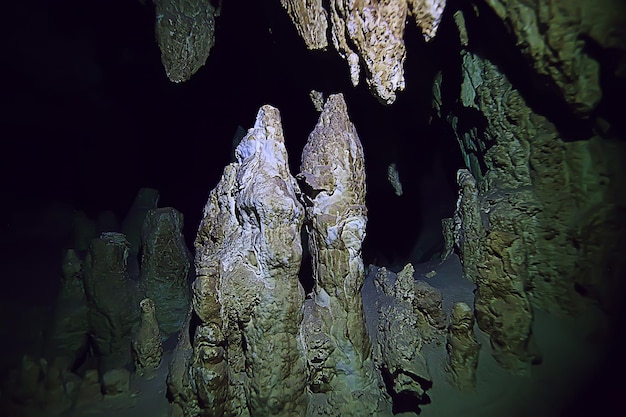The image displays a captivating underground scene set within a dark cave, emphasized by a black background that engulfs the surroundings. Dominating the foreground are stalagmites, which are pointy rock formations rising from the cave floor. They vary in size, with some being short and others notably taller, and are composed of various shades of white, gray, and green, giving them a textured, knobby appearance reminiscent of wood. Above these are the stalactites, hanging precariously from the cave ceiling in hues of brown, cream, white, green, and gray. These formations are created over hundreds of years by mineral-rich water dripping and depositing layers of sediment. The dimly lit environment creates an eerie yet fascinating atmosphere, with larger formations protruding upward and in the middle, flanked by smaller ones on either side. The scene also hints at deeper, unseen sections of the cave, shrouded in darkness, inviting further exploration.